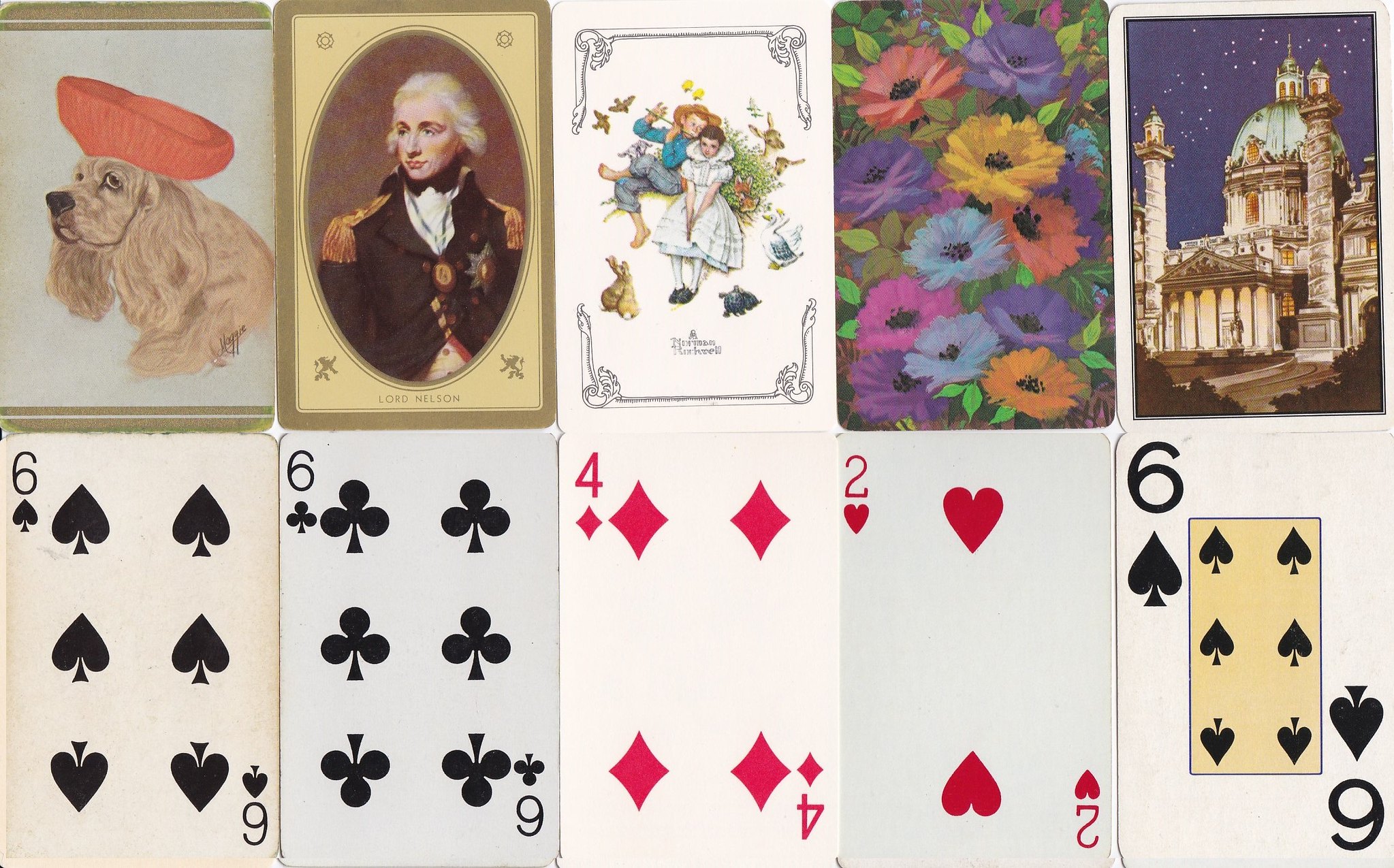This image showcases an array of playing cards, meticulously arranged in two rows. The upper row features the elaborate designs on the backs of five cards, presented from left to right. The first card displays an adorable illustration of a dog wearing a red hat. The second card depicts a distinguished figure in an oval frame, adorned in a white wig and a military uniform. The third card appears to draw inspiration from a fairy tale, portraying what seems to be the Pied Piper as a child in a white dress, accompanied by a male figure clad in rolled-up jeans and a straw hat, playing a pipe. The fourth card is a vibrant display of flowers in gold, purple, and blue hues. The final card in this row shows an imposing government building with domes and columns, framed against a night sky.

The bottom row consists of five cards aligned directly beneath those in the top row, revealing their faces instead of their backs. From left to right, these cards are the six of spades, six of clubs, four of diamonds, two of hearts, and another six of spades. These cards exhibit traditional designs, with black suits (spades and clubs) on white backgrounds, and red suits (diamonds and hearts) on white backgrounds. Notably, the shades of white on the cards' backgrounds vary subtly, adding an extra layer of detail to the overall composition.